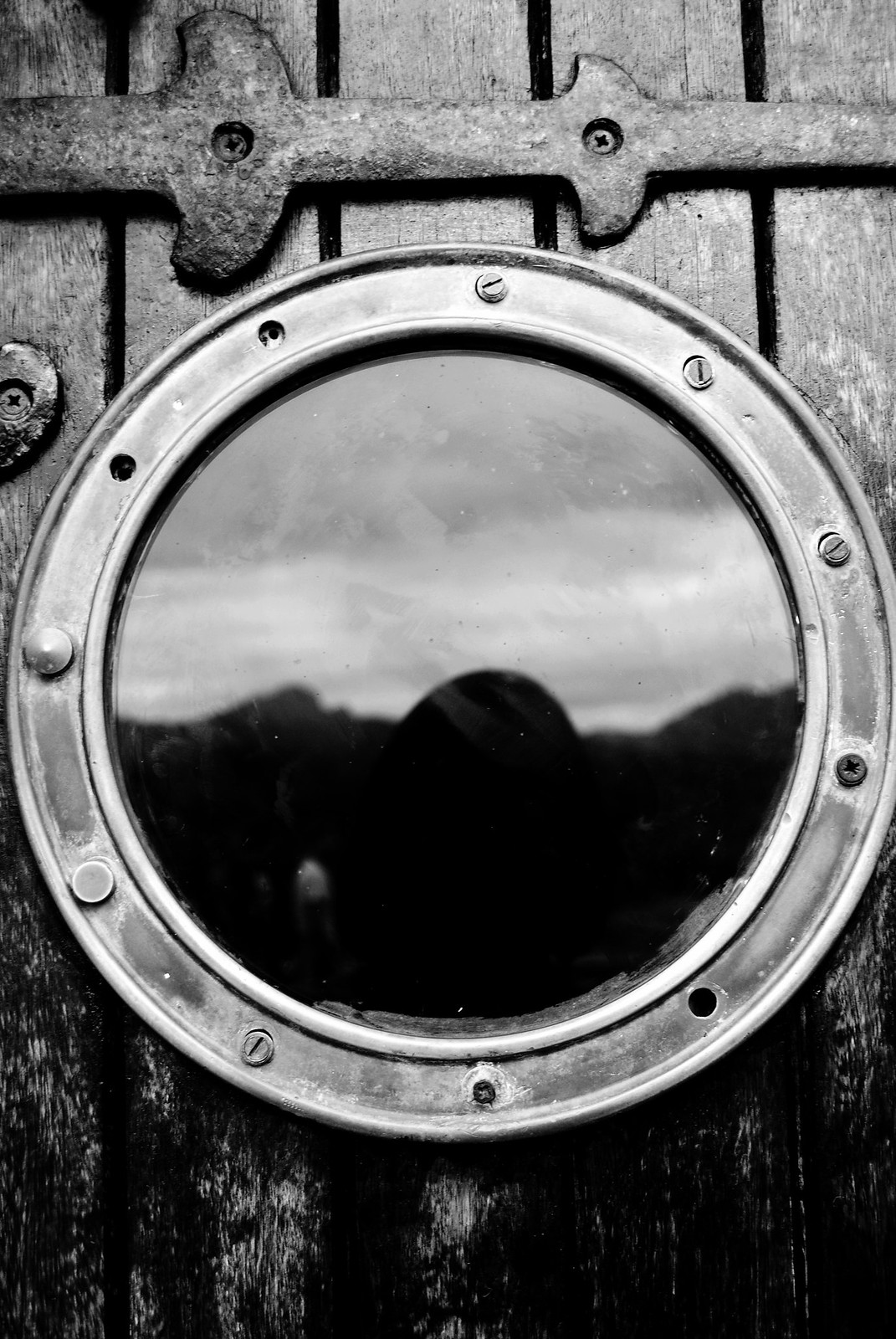This black-and-white close-up photo captures a round porthole window, reminiscent of those found on ships or boats, firmly secured to a wooden surface by an array of rivets and bolts. Specifically, the window is encircled by approximately 10 to 12 bolts, although some bolts appear to be missing. The glass of the porthole provides a reflection of the outside environment: the upper part of the reflection reveals a gray, cloudy sky, while the lower part displays a dark, curved shape resembling distant hills or mountains. The window is affixed to vertical wooden slats that appear weathered, particularly along the bottom edge, suggesting long-term exposure to the elements, possibly even submersion underwater. Additionally, a horizontal metal bar, fastened with two Phillips screws, spans the wooden slats just above the porthole, adding to the structural detail of the scene.